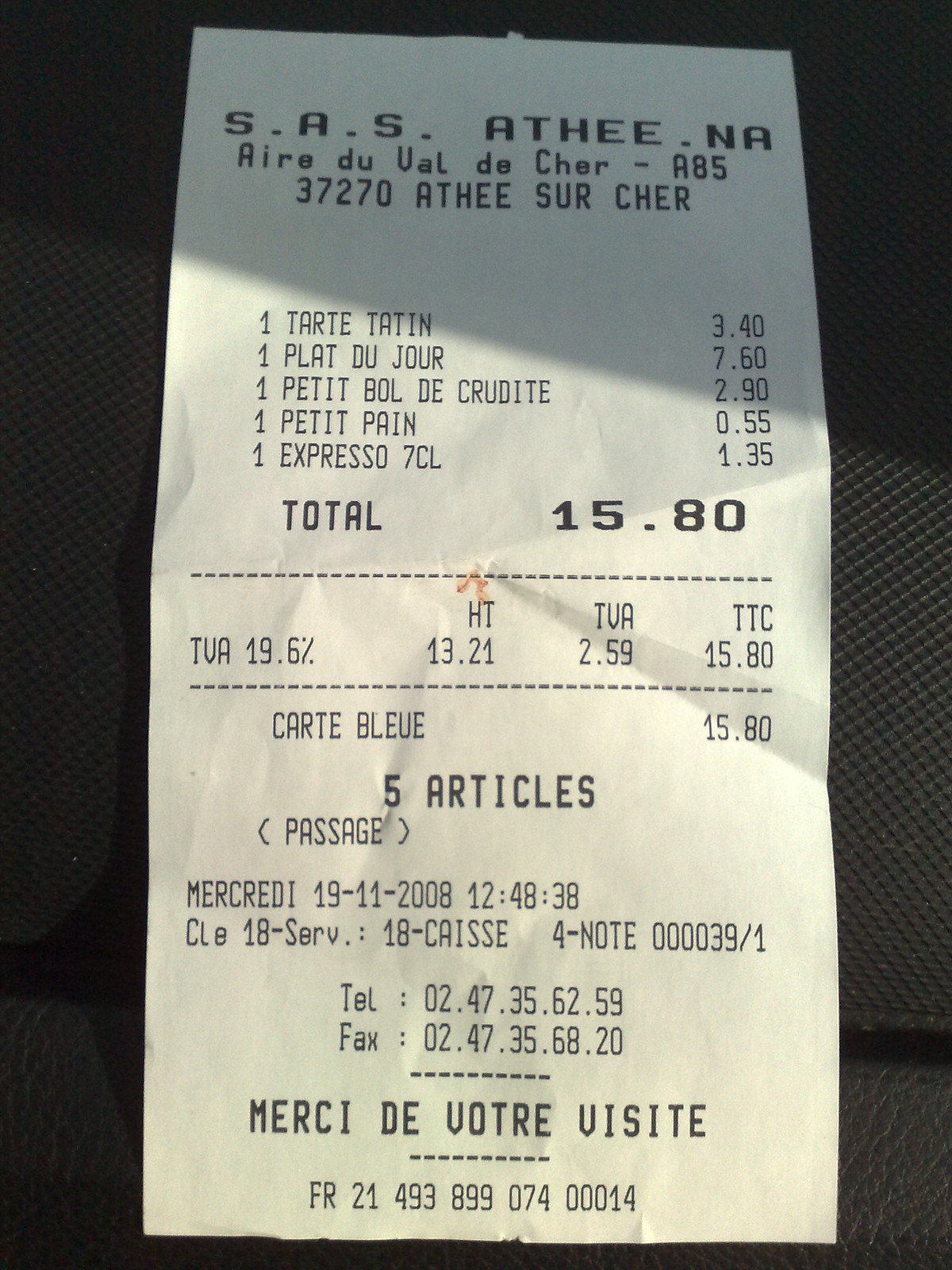The image features a white receipt resting on a black upholstery surface, possibly a car seat or dashboard. The receipt, written in French, details five items purchased, with individual prices of $3.40, $7.60, $2.90, $0.50, and $1.35, totaling to $15.80, likely in Euros. The receipt is partially illuminated by sunlight, which enhances the contrast against the darker background. At the top, the retailer is identified as "S-A-S-A-F-E dot N-A." The bottom of the receipt lists contact information, including a telephone number (02.47.35.62.59) and a fax number (02.47.35.68.20), along with the phrase "Merci de votre visite," translating to "Thank you for your visit." The date on the receipt is from 2008.